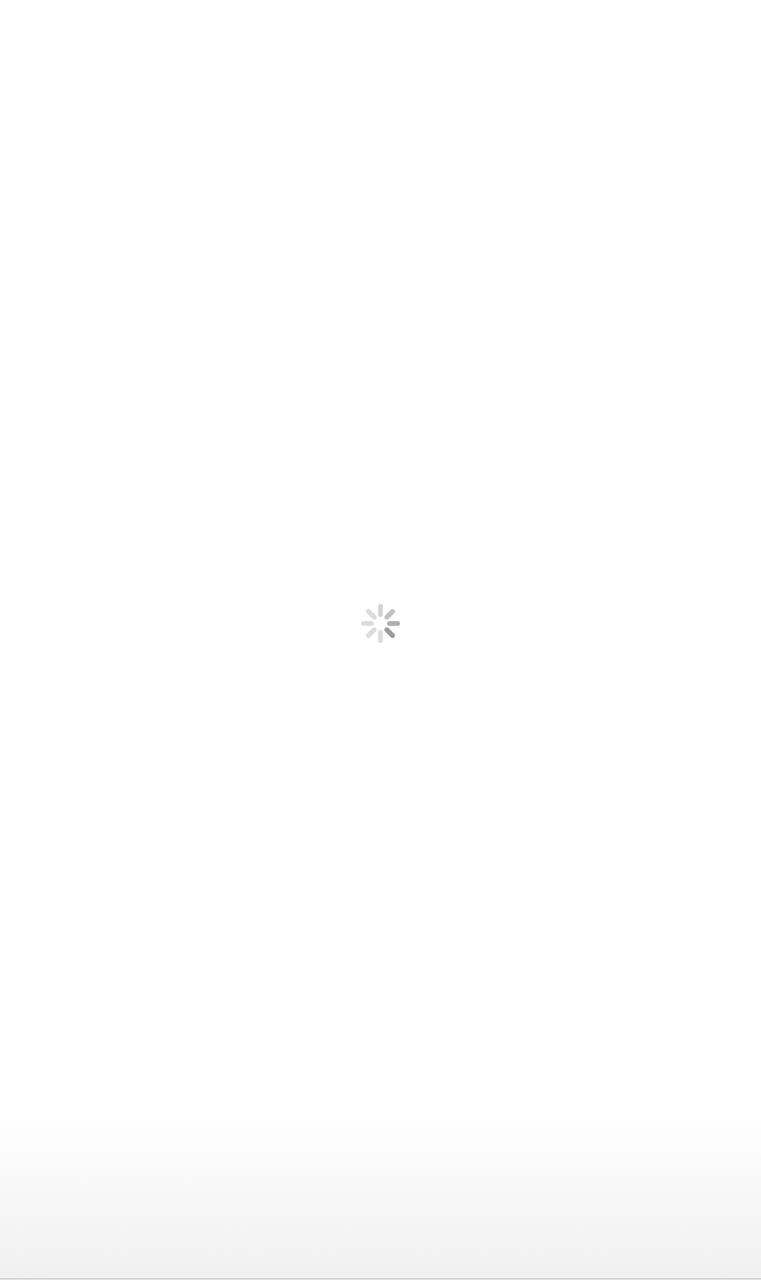This is a screenshot of a nearly all-white webpage, creating an effect that makes it difficult to discern the image’s size at the top as it blends seamlessly with the background of the page. Dominating the lower portion of the image is a centrally-located gray circular loading icon, indicative of a page or media content that is in the process of loading. Apart from this, the image is devoid of any colors, text, or other distinguishing features. Additionally, there is a subtle, light gray band approximately two centimeters in height running across the very bottom of the image. The overall composition conveys a sense of incompleteness and anticipation, typically associated with loading screens.